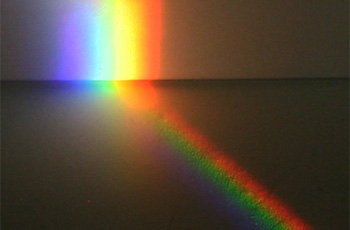This is a small rectangular image depicting the dimly lit edge of a room where the floor meets the wall. The ambient light is very low, resulting in a predominantly dark brown background that gradually transitions into a lighter shade towards the top. At the center of the image, cutting diagonally from the lower right corner to the upper left, is a striking beam of light, presumably cast through a prism. This beam creates a vibrant rainbow pattern both on the floor and along the wall. On the floor, distinct red and green beams extend from the bottom right, gradually merging into a spectrum of colors closer to the wall. Upon reaching the wall, the light spreads out, revealing a full spectrum array from red through orange, yellow, green, blue, and purple. The most vivid parts of the spectrum are projected vertically along the wall and slightly onward from the point where the floor and wall converge. The contrast between the dark surroundings and the colorful prism light forms a captivating visual composition, highlighting the vivid colors red, green, blue, yellow, orange, and purple, which starkly stand out against the otherwise dark scene.